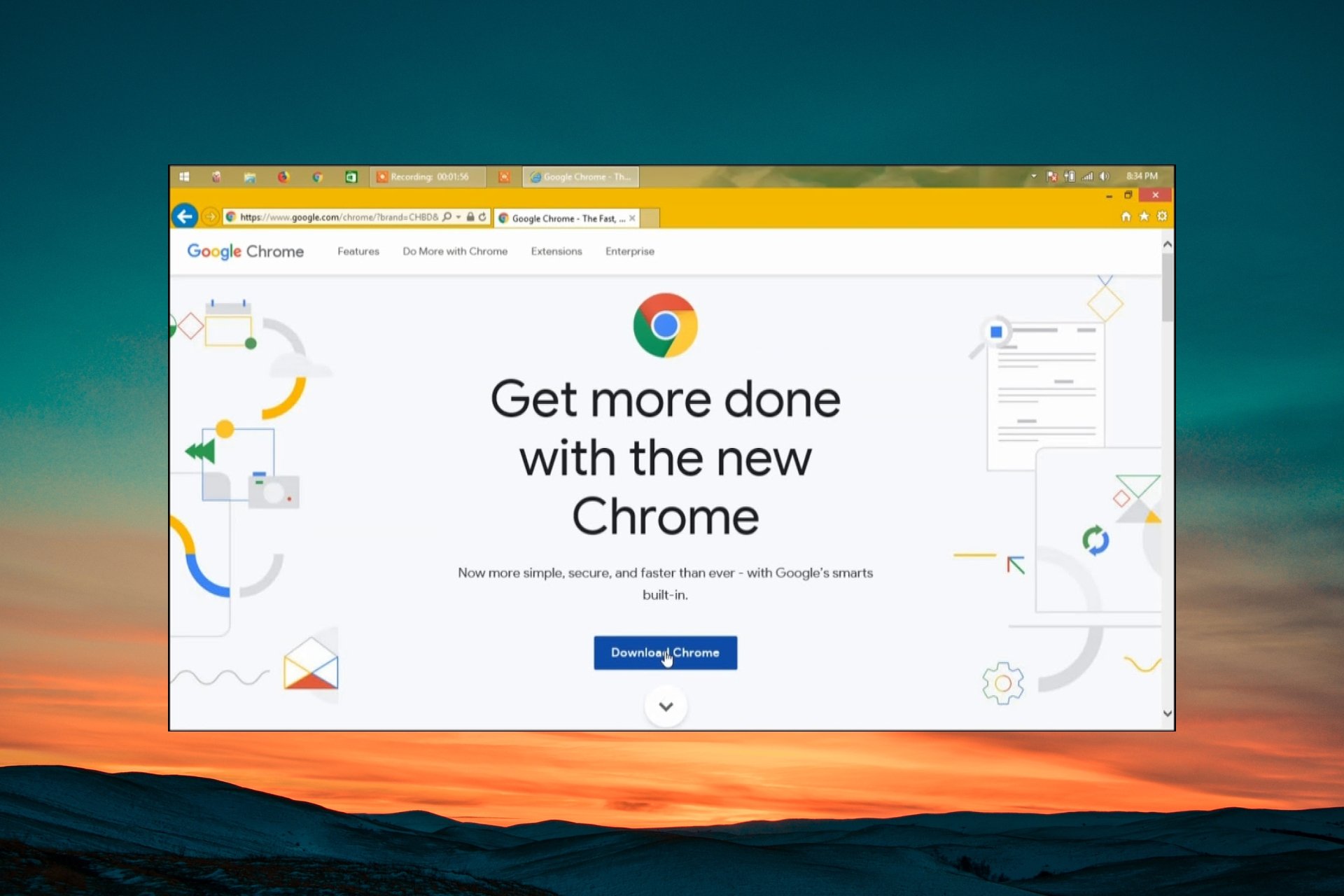The image features a screenshot superimposed on a serene sunset background. The sky transitions from a dark blue at the top to a vibrant orange near the horizon, where dark silhouettes of hills are visible. The centerpiece of the image is a screenshot from a web page with a URL displayed as "https://www.google.com" in the search bar. The banner at the top of the page includes tabs labeled "Google Chrome features," "Do more with Chrome," "Extensions," and "Enterprise." Prominently in the middle, a message reads: "Get more done with the new Chrome. Now more simple, secure, and faster than ever with Google's smarts built in. Download Chrome." A hand icon hovers over the "Download Chrome" button, suggesting an interactive element. There are no visible people, animals, plants, buildings, vehicles, bicycles, or birds in the image, creating a clean and focused visual composition.